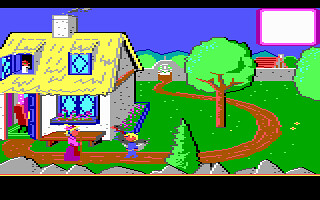The image depicts a scene from a computer game under a dark blue sky. In the upper right corner, there is a white rectangular notification with a pink frame. Dominating the left side of the picture, nearly reaching the middle, is a partially cut-off house viewed from the front. The house features an open door with a person walking through. To the right of the door, two windows are adorned with flower beds. The second floor of the house is painted yellow, and it appears to be the roof level. On this floor, there are two windows; the window on the left is open and someone is peering out.